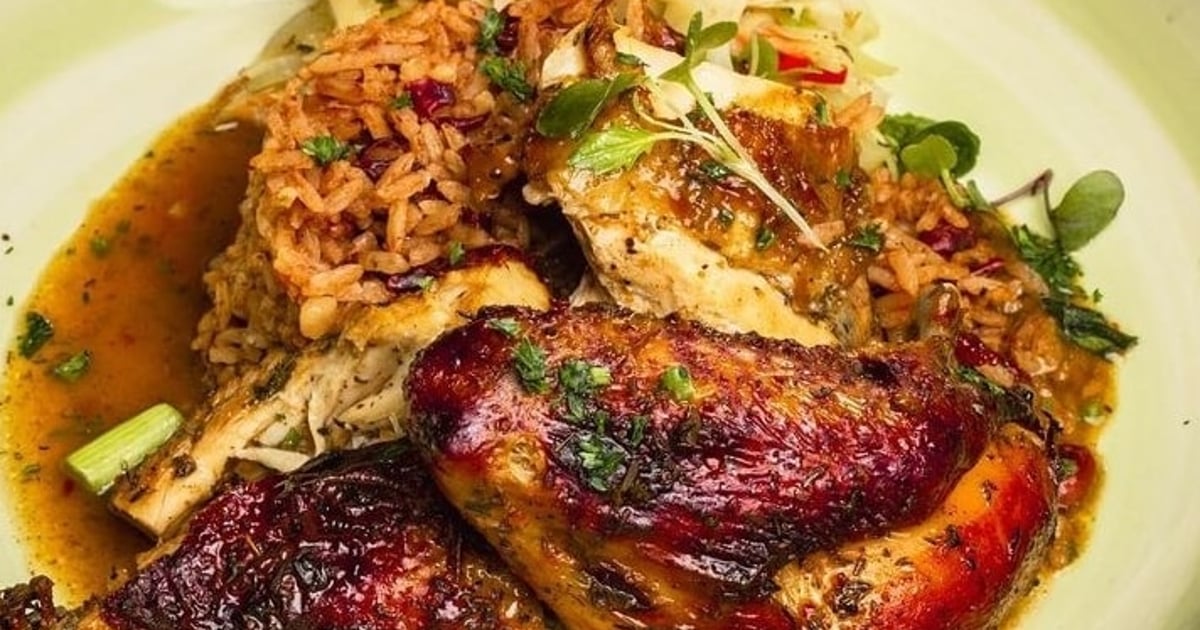This is a close-up photograph of a meal served on a circular white plate with a greenish border. The central focus is a large portion of what appears to be either chicken breast or turkey, garnished with chopped green onions and possibly chives. The bottom half of the plate is predominantly occupied by this meat. On the top half of the plate, there is a serving of brown, oval-shaped rice mixed with beans and peppers, giving it a spicy flair. The rice is seasoned with orange highlights and further garnished with green herbs, adding a touch of elegance to the dish. Nestled among the rice is a sprig of possibly parsley, contributing to its visual appeal. A brown sauce pools in the center of the plate, blending with the green onions and other greens, likely enhancing the overall flavor of the meal. A few loose green leaves are scattered in the upper right corner of the plate, completing the presentation. The photograph focuses solely on the food and plate, with no distinguishable background, delivering an intimate, albeit unrefined, view of the dish.